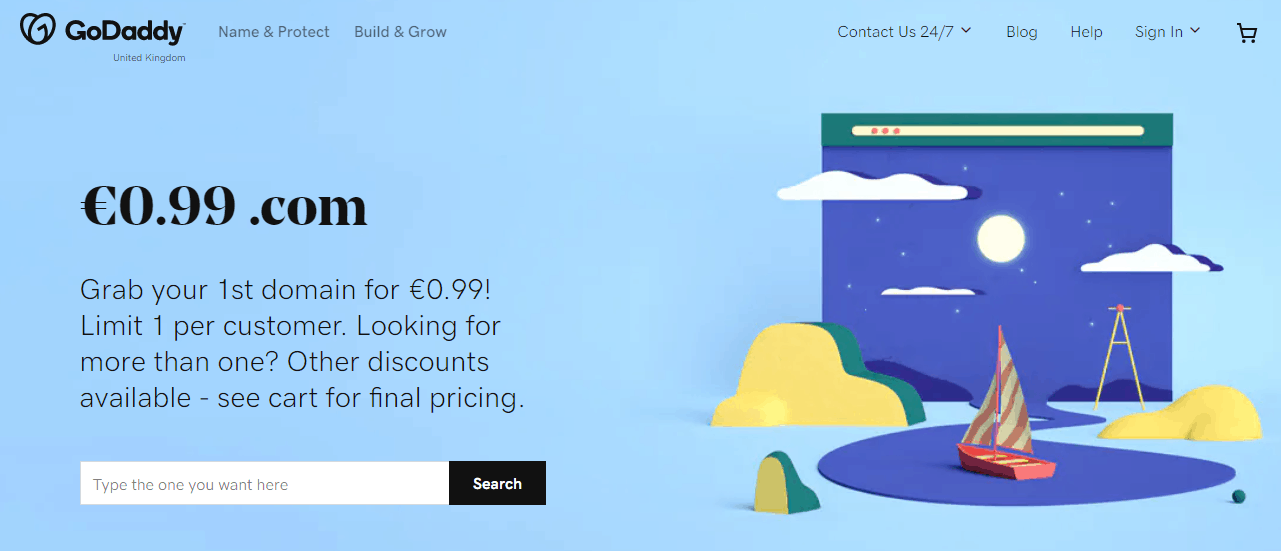The screenshot captures the GoDaddy homepage with a clean and organized layout. At the top left corner, "GoDaddy" is prominently displayed in bold black text, accompanied by the GoDaddy logo resembling a stylized heart, also in black. Adjacent to the site name, two primary categories are visible: "Name & Protect" and "Build & Grow." 

On the top right of the image, a shopping cart icon is nestled, indicating the online store feature. To its left are additional navigational options: "Sign In" with a downward arrow, "Help," "Blog," "Contact Us 24/7" with a downward arrow beside it, offering various customer assistance options.

Dominating the middle-left section of the image is a promotional message: "99cents.com. Grab your first domain for 99 cents. Limit one per customer. Looking for more than one? Other discounts available. See cart for final pricing." Below this promotional text, a search bar invites users to "type the one you want here," with a black box to its right inscribed with the word "Search" in white text.

The right side of the image displays artistic depictions that suggest a website interface with a serene sky background featuring blue skies, fluffy clouds, and a moon, indicative of GoDaddy’s web design and hosting services.